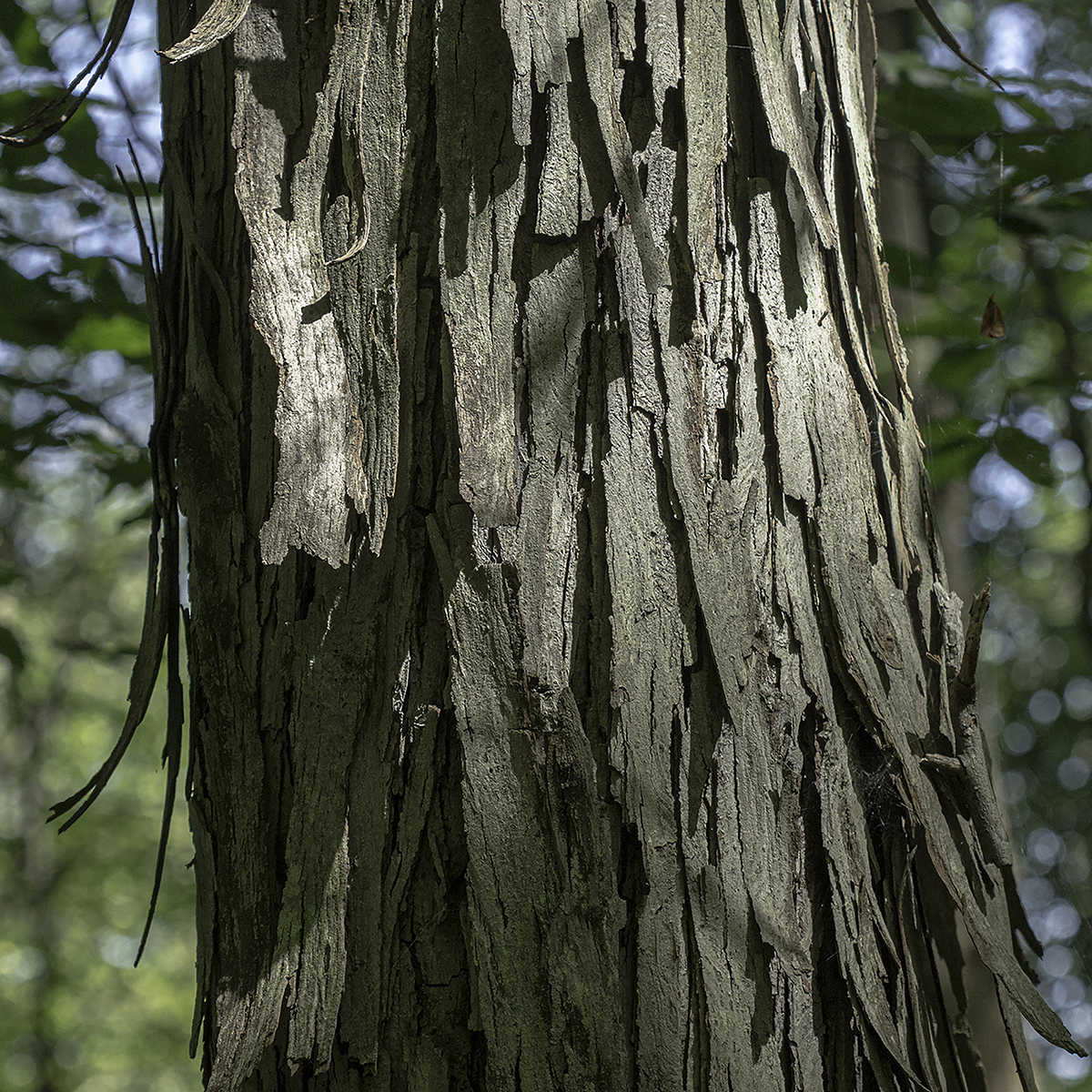The image is a close-up photo of a tree trunk with peeling bark. The bark, which is grayish to dark gray and slightly charcoal in color, consists of narrow, long strips that are loosely attached and curling outward, creating a rough and uneven texture. In the background, there is a faint, blurry presence of greenery and leaves, suggesting the tree is situated within a forest. The lighting in the image illuminates the right side of the tree trunk, while the left side remains in shadow. The tree trunk, positioned centrally from top to bottom, is the clear focus of the image, highlighting the intricate details of its peeling bark.